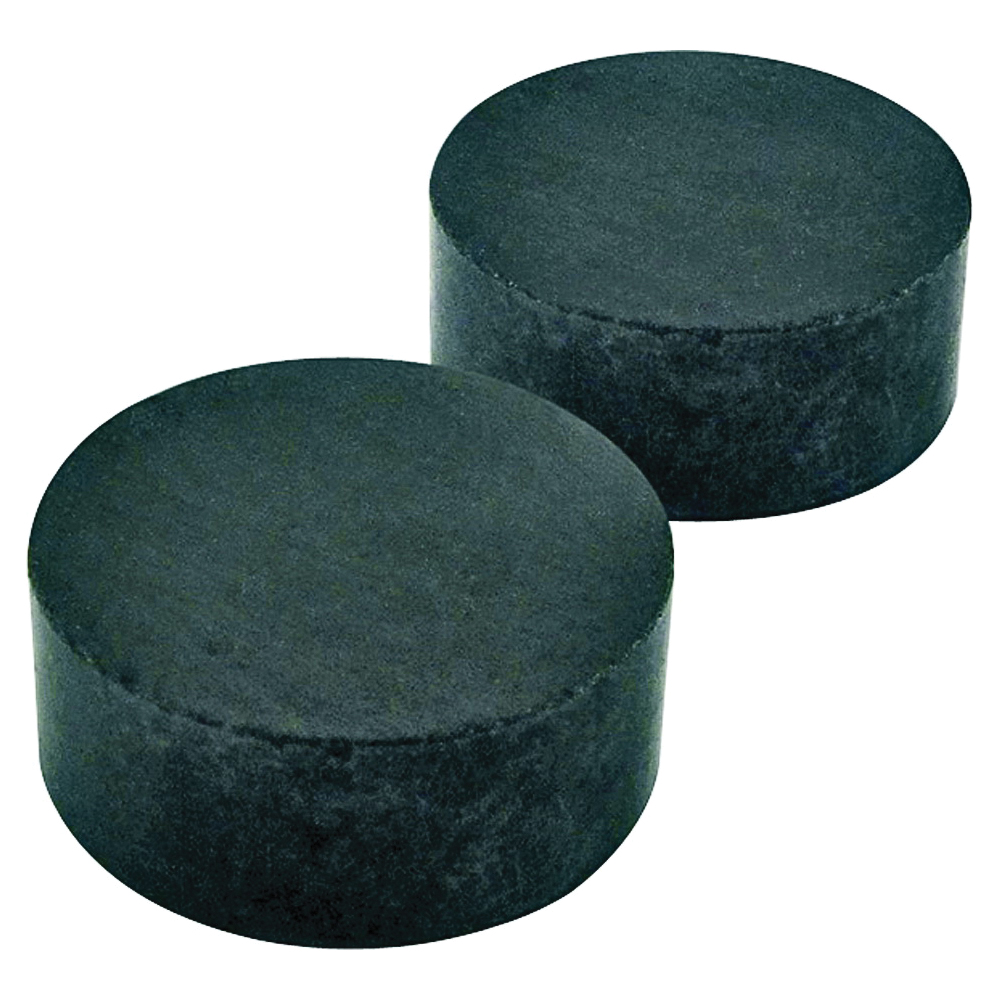The image features two black, cylindrical objects that strongly resemble hockey pucks, positioned diagonally with one on the bottom left and the other above it to the top right. These disk-shaped items, equally sized and shaped, exhibit slight wear along their edges. The background is a solid white, accentuating the dark objects that have flat tops and bottoms. There is no text, labels, or numbers in the photograph. Despite alternative interpretations, such as them being fabric-covered items like ottomans, the uniformity in size and shape, along with the color and cylindrical form, suggests the objects are most likely well-worn hockey pucks rather than any type of furniture.